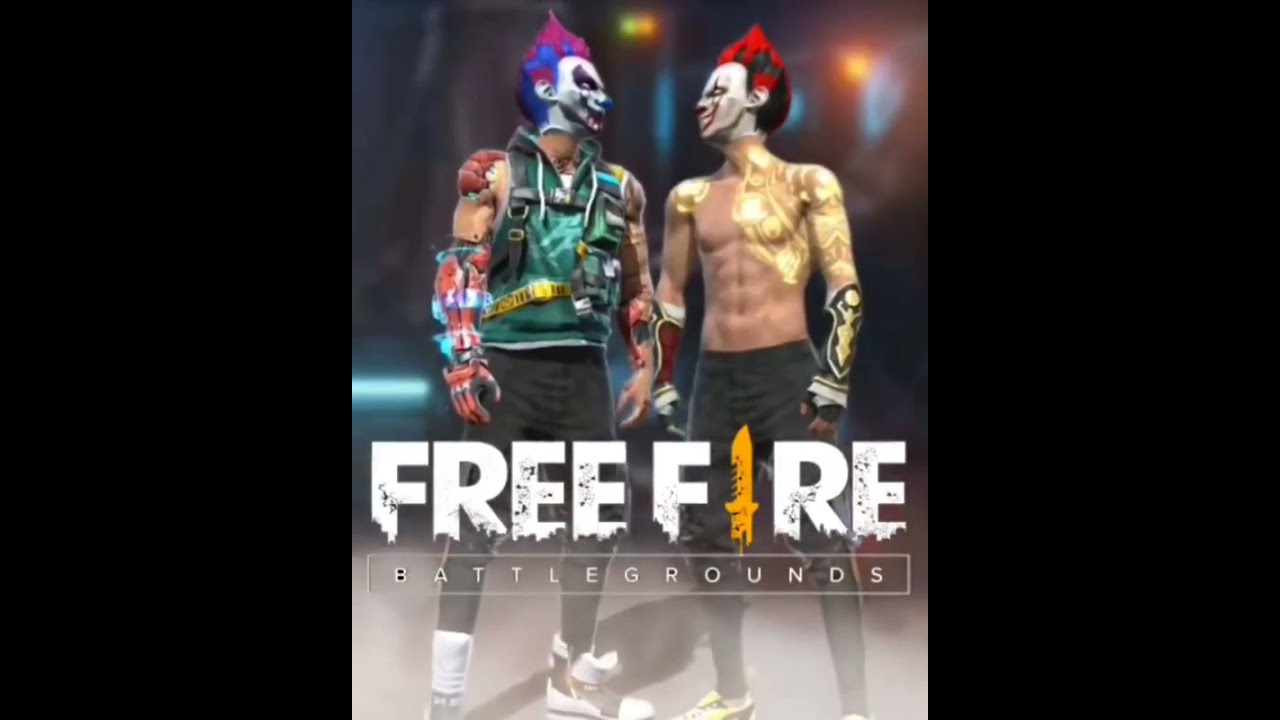The image is a screenshot of an advertisement for a video game called "Free Fire Battlegrounds." Prominently displayed at the bottom center of the image is the game's title, where "Free Fire" is rendered in white text with a unique, grungy appearance—chunks missing from the bottom of the letters and black specks scattered across them. The "i" in "fire" stands out as it resembles a yellow knife or sword. Below the main title, in a thin gray rectangle, the word "Battlegrounds" is written in gray text.

In the background, the scene is a blend of fluorescent green and orange lights, providing a dynamic, blurry backdrop. Two distinct 3D game characters are featured prominently. 

On the right side is a menacing character without a shirt, sporting black pants. His chest and arm bear gold paint, resembling intricate tattoos or body art, and he wears gloves that extend up to his wrists. His upper arm is adorned with a black and gold braced piece, and his face is strikingly painted white. His hair, mostly black, has a red top.

The character on the left has similarly sinister vibes, with a white painted face and spiky hair colored in pink and blue. He is clad in a green shirt topped with a vest featuring black straps and a possible parachute harness. His heavy, orange, white, and teal gloves extend past his elbows. He wears black pants paired with white shoes that rise above his ankles.

This highly detailed and visually arresting advertisement captures the intense and chaotic atmosphere of "Free Fire Battlegrounds."